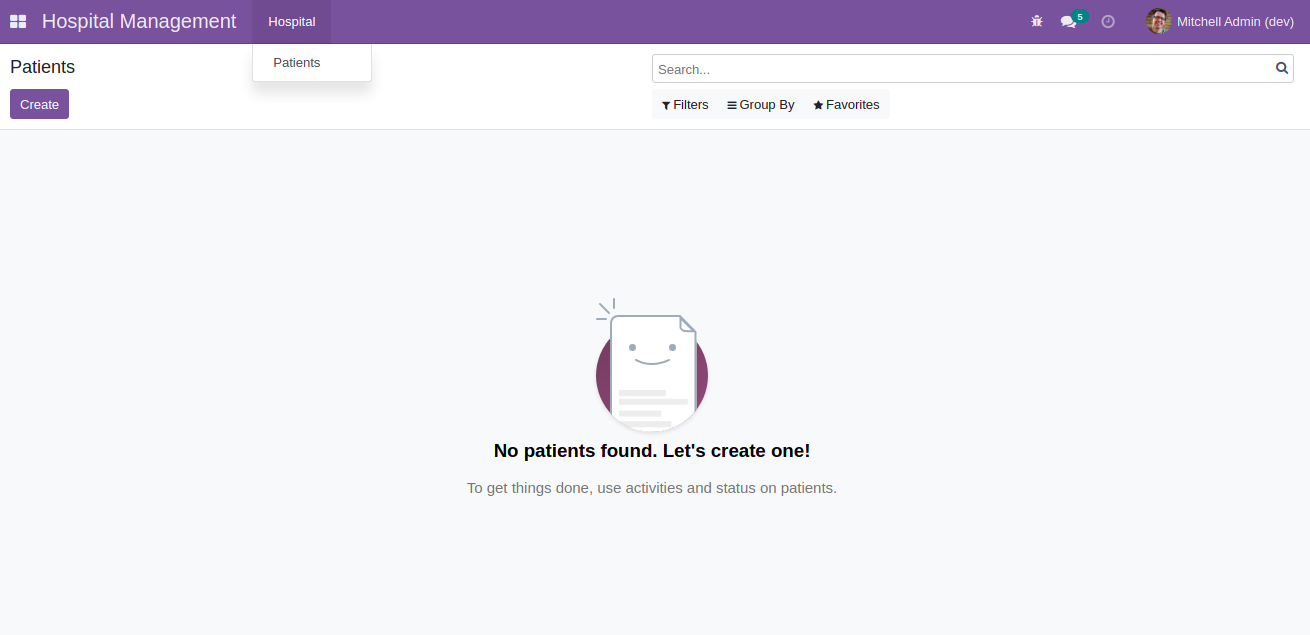Here's a detailed and cleaned-up description for the image:

---

The image is a screenshot from what appears to be a website or an app interface. The background is predominantly white, featuring a prominent purple navigation bar at the top. On the left side of this bar, "Hospital Management" is inscribed in white text, accompanied by a window icon. Slightly to the right, the word "Hospital" appears with a small drop-down arrow and the word "Patients" beneath it. 

On the far right of the purple bar, there are several icons. A speech bubble icon, which possibly indicates messages, shows the number "6" in green, although the exact number is a bit unclear. Adjacent to this is an icon representing a person, labeled "Mitchell Admin Dev."

Below the navigation bar, on the left side of the screen, the word "Patients" is written in black. Directly underneath, a purple button labeled "Create" invites the user to add new patient information. To the right of this button is a search box, accompanied by the text "Filters," "Group by," and "Favorites," each with small black icons to their left.

Centered on the lower part of the page is a stylized cartoon illustration of a piece of paper with eyes and a smiling face. Three lines emanate from the left edge of this cartoon figure, while the top right corner is artistically folded. Below this paper-like figure, there are several gray horizontal lines intended to represent text.

Purple semicircles are faintly visible on the left and right edges of the screen. Beneath the illustration, in the center, is a black text message stating, "No patients found. Let's create one."

Further below, a secondary message suggests using activities and status on patients to manage tasks, though it humorously acknowledges the implausibility of a hospital having no patients.

---

This caption is crafted to be detailed and clear, helping a reader to visualize and understand the image thoroughly.